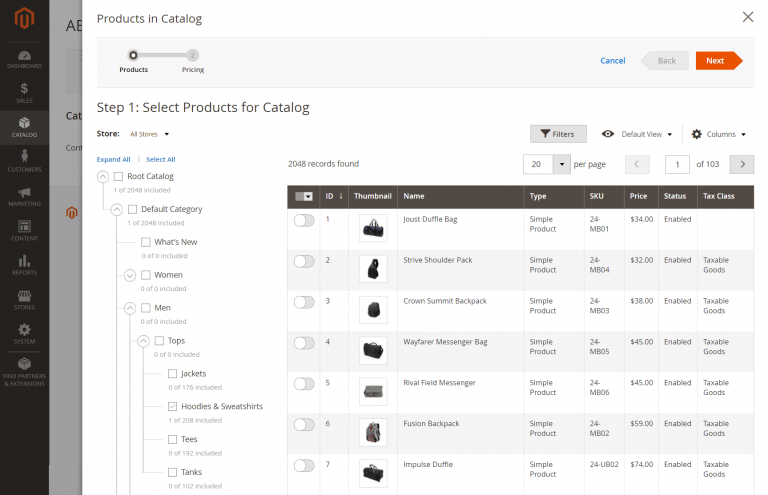At the top of the screenshot, the menu displays "Products and Catalog." A toggle switch is shown, with the current setting on "Products" rather than "Pricing." To the right, buttons for "Cancel," "Back," and "Next" are visible. This is Step 1, which involves selecting products for the catalog.

The store settings section follows, showing options such as "Store: All Stores," "Expand All," "Select All," and "Root Catalog." Specific categories within the catalog are listed with details on the number of items included:

- "Default Category": 1 of 2048 included
- "What's New": 0 of 0 included
- "Women": 0 of 0 included
- "Men": 0 of 0 included
- "Tops": 0 of 0 included
  - "Jackets": 0 of 176 included
  - "Hoodies and Sweatshirts": checked, with 1 of 208 included
  - "Tees": 0 of 192 included
  - "Tanks": 0 of 102 included
  
To the right, it shows there are "2048 Records Found," with a display setting of "20 per page," currently showing page "1 of 103." Detailed information for seven products is listed:

1. **Joust Duffel Bag**
   - Type: Simple Product
   - SKU: 24-MB01
   - Price: $34
   - Status: Enabled
   - Tax Class: Left Blank

2. **Strive Shoulder Pack**
   - Type: Simple Product
   - SKU: 24-MB04
   - Price: $32
   - Status: Enabled
   - Tax Class: Taxable Goods

3. **Crown Summit Backpack**
   - Type: Simple Product
   - SKU: 24-MB03
   - Price: $38
   - Status: Enabled
   - Tax Class: Taxable Goods

4. **Wayfair Messenger Bag**
   - Type: Simple Product
   - SKU: 24-MB05
   - Price: $45
   - Status: Enabled
   - Tax Class: Taxable Goods

5. **Rival Field Messenger**
   - Type: Simple Product
   - SKU: 24-MB06
   - Price: $45
   - Status: Enabled
   - Tax Class: Taxable Goods

6. **Fusion Backpack**
   - Type: Simple Product
   - SKU: 24-MB02
   - Price: $59
   - Status: Enabled
   - Tax Class: Taxable Goods

7. **Impulse Duffel**
   - Type: Simple Product
   - SKU: 24-UB02
   - Price: $74
   - Status: Enabled
   - Tax Class: Taxable Goods